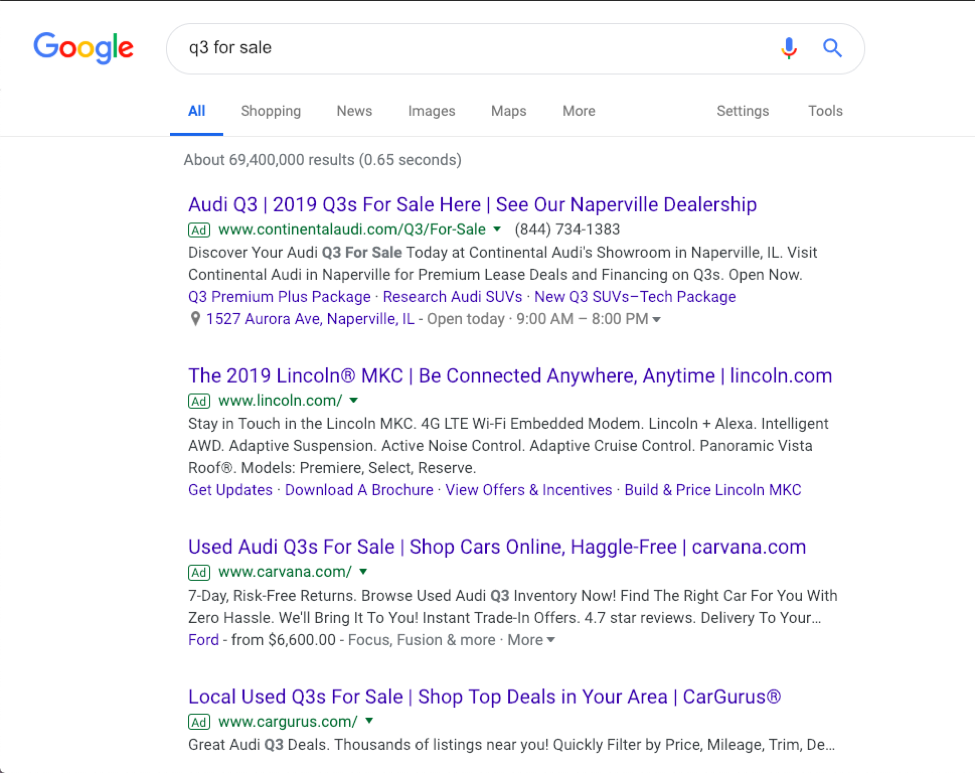The image displays a Google search results page in the classic white theme with the iconic rainbow-colored Google logo positioned in the upper left corner. In the central search bar, the query "Q3 for sale" has been entered. Adjacent to this search bar on the right, a blue and red microphone icon can be seen, signifying voice search capability, along with a blue magnifying glass icon for search functions.

Below the search bar, the standard set of Google search categories is visible. The 'All' category is currently selected, evidenced by its blue text and underline, whereas categories like 'Shopping,' 'News,' 'Images,' 'Maps,' and 'More' are in gray, indicating they are not active.

The cropped screenshot captures the top four search results, all of which are advertisements. Each ad features a blue clickable link, primarily related to the Audi Q3, except for one entry listing a 2019 Lincoln MKC. The ads display URLs in green, sourced from websites such as Continental Audi, Lincoln.com, Carvana.com, and Cargurus.com. Next to each URL, a green label with "Ad" confirms their promotional nature.

These ads are accompanied by metadata snippets in black text, giving brief descriptions of the offerings. Some entries have additional quick links below, providing options like "Q3 Premium Plus package," "Get updates," or "Download a brochure." The top-listed ad uniquely includes a phone number for direct inquiries.